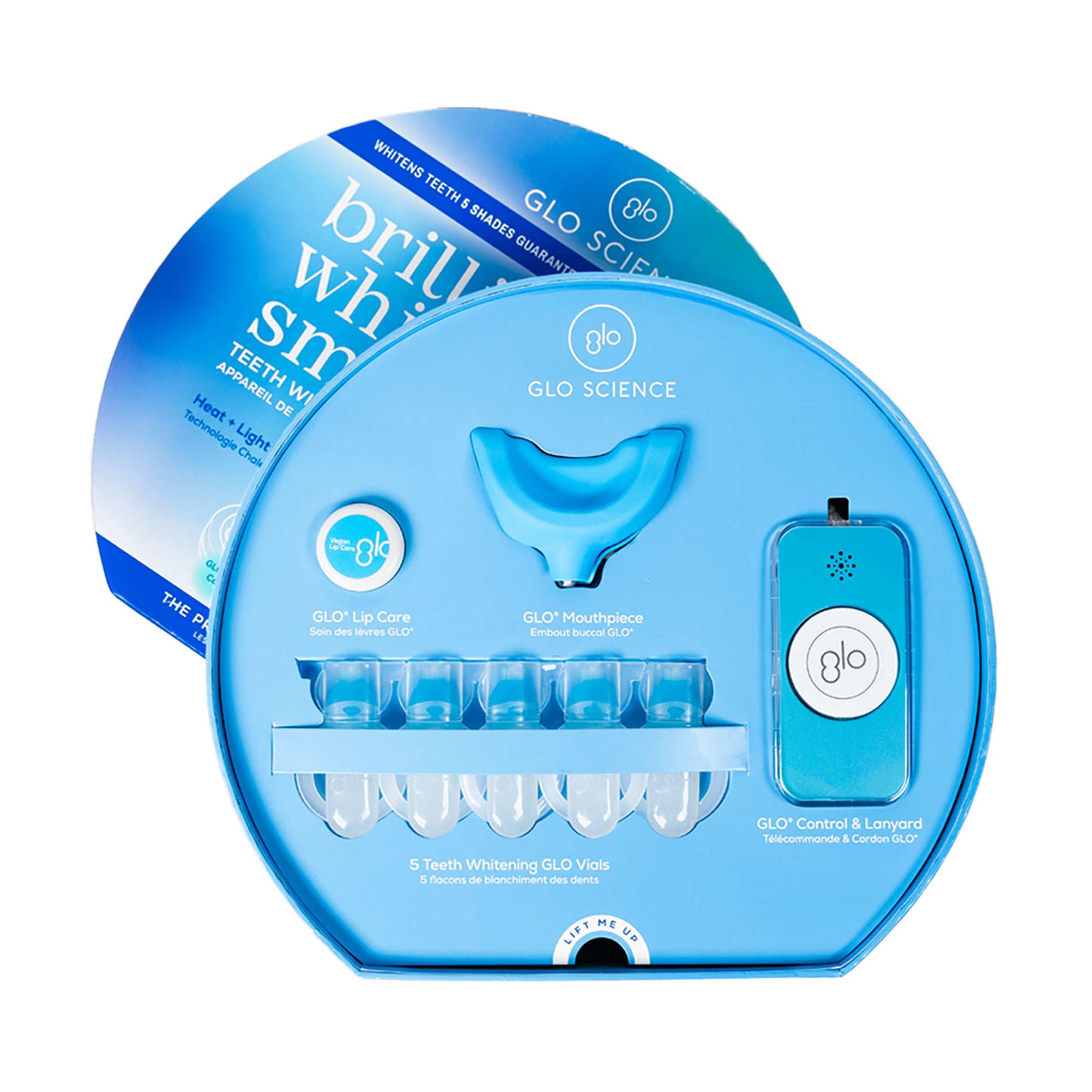The image depicts an advertisement for a teeth whitening product called Glow Science. The centerpiece is an almost circular tray with a flat bottom for stability, prominently featuring the "Glow Science" branding and a GLO logo in a circle. The kit includes a blue Glow Mouthpiece for administering the whitening treatment. Accompanying this are five teeth-whitening glow vials, which are used to fill the mouthpiece. Additionally, there is a tub of Glow Lip Care, likely lip balm, positioned to the left. To the right, there is a Glow Control and Lanyard, resembling a small device with a prominent button in the middle, which might be used to activate the light and heat mechanism suggested by the label "Light Me Up". Behind the main product is the partially visible outer packaging, emphasizing the brand's promise of a progressively brilliant white smile. The product design showcases an appealing palette of medium blue, light blue, and white, enhancing its visual appeal.